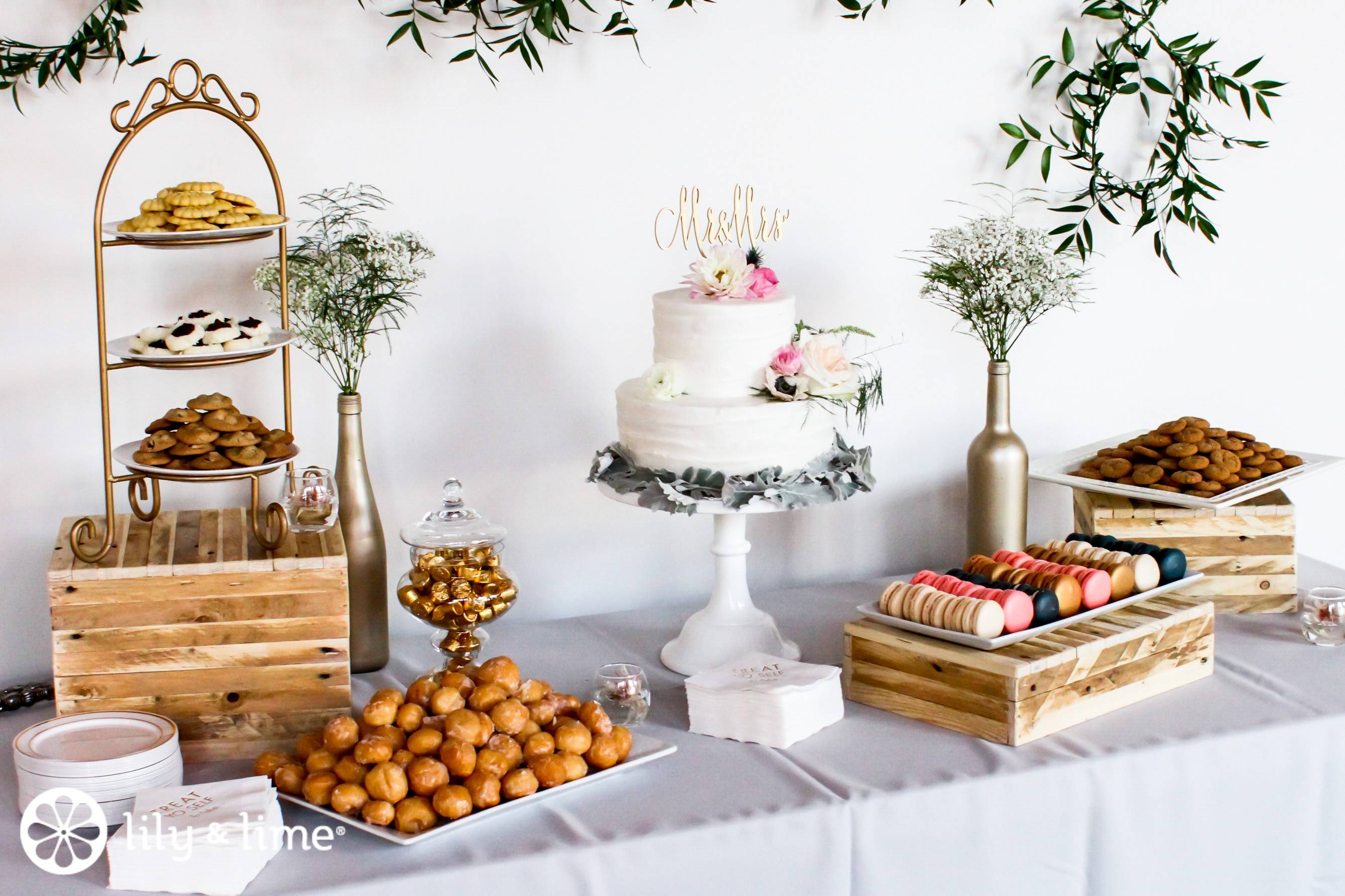The image captures a professional, full-color, horizontally rectangular photograph of a beautifully curated wedding reception table set up by a catering company. The table, draped in a pristine white tablecloth, is situated indoors against a white wall with a discrete name tag in the lower left-hand corner reading "Lily and Lime." 

At the center of the display stands a majestic two-tiered white wedding cake adorned with a "Mr. and Mrs." topper, placed on a pedestal plate. To the right of the cake, a tray showcases a colorful array of cookies including shades of beige, pink, dark blue, and brown. To the far right, a square tray holds a darker-colored treat, likely chocolate, and is complemented by a vase of baby's breath acting as a simple yet elegant decorative element.

On the left side of the table, a three-tiered display of assorted cookies is elevated on a wooden box, showcasing brown cookies and a variety of other types. Further to the left, a large tray presents an abundance of donut holes. This beautifully styled wedding table exudes an inviting and celebratory atmosphere, highlighted by the thoughtful arrangement of sweet treats and decorative greenery.